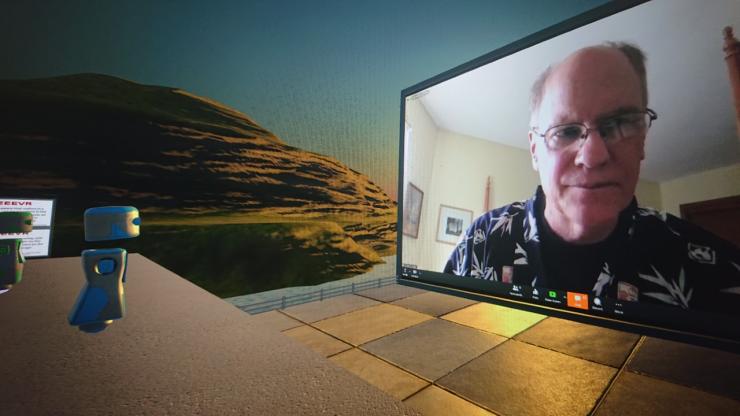In a surreal computer-rendered scene, two small robots with floating, disc-shaped heads and segmented metal bodies stand on a raised concrete platform on the left side. One robot is blue, and the other is green. To the right, a tiled floor is enclosed by a blue fence. In the distance, beyond the fence, a computer-generated green and brown mountain rises against a blue sky with the sun setting behind it. Dominating the background, a large flat-screen display, reminiscent of a drive-in movie theater screen, shows an older Caucasian man with glasses and thinning hair. He wears a navy blue Hawaiian shirt over a black t-shirt and appears to be in a room with white walls, looking off to the right as if captured during a Zoom call. The robots seem to be either observing or interacting with the content on this enormous screen, blending elements of a virtual landscape with a touch of futuristic interaction.